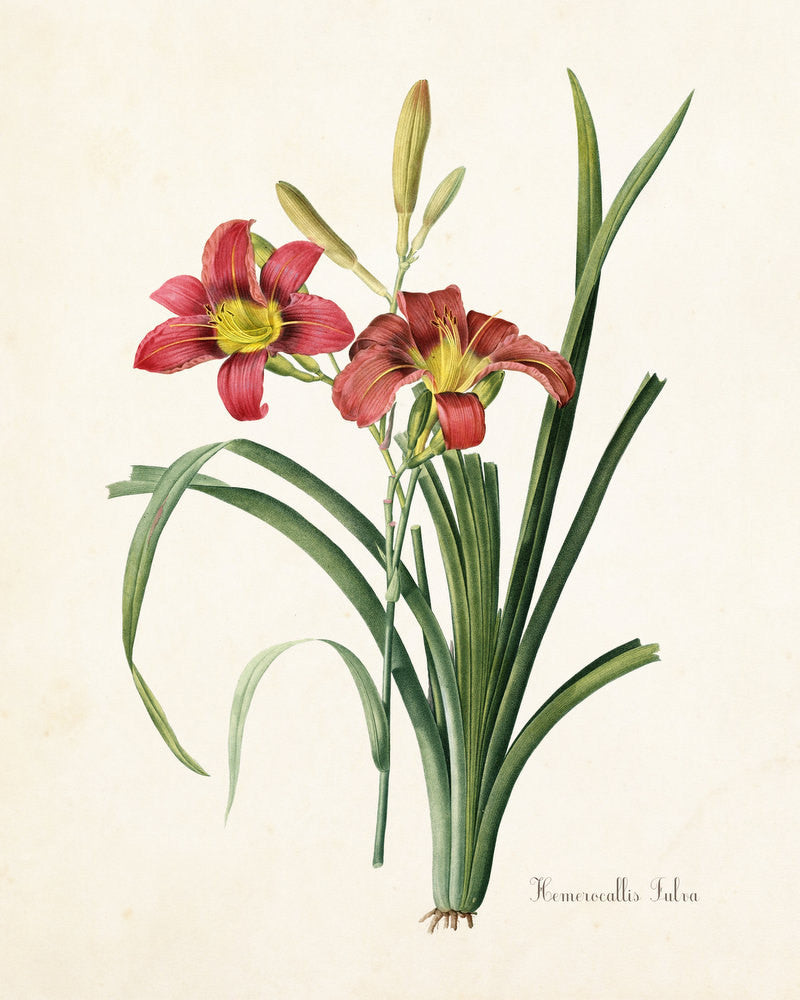This botanical illustration depicts a vibrant red lily, labeled in cursive in the lower right corner as "Hemerocallis fulva." The flower garners attention with its striking six-petaled blooms where the red outer petals transition seamlessly into a yellow center. The long stamens, reaching out from the center, are tipped with brown, adding to the intricate details. The plant features several tall green stems with accompanying leaves that descend from a darker green at the base to a lighter hue at the tips. Additionally, the artwork captures several greenish-yellow buds at various stages of opening. The illustration is set against a cream background, making the vivid colors of the lily stand out. Tiny brown roots are noticeable at the bottom of the plant, grounding the detailed botanical study.